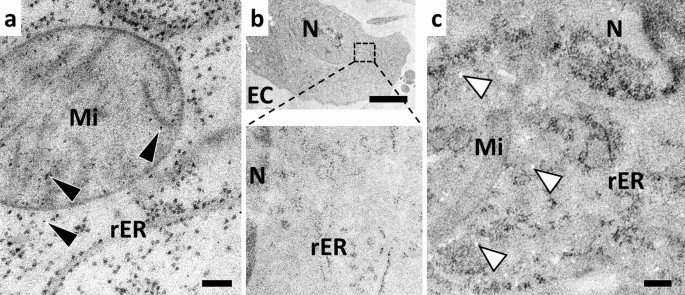The image consists of three black and white satellite photographs labeled A, B, and C. Each photograph appears to depict different terrain features, possibly geological or man-made structures marked with various letters and symbols. 

**Image A** shows a slightly hilly terrain with the letters "MI" superimposed over the top. Below, the text "RER" is written in black, and there are three triangular arrows pointing leftward, located on the bottom left, above that to the right, and then to the upper right of that particular arrow. In the bottom right is a small black dash.

**Image B** portrays terrain that may include a hill or lake, with the letter "N" marked at the top. The bottom part of this image includes the text "EC" on the bottom left and "RER" along the center, separated by a dotted line into different segments. The lower right contains a small black dash.

**Image C** shows lightly wooded terrain with shrubs. The top right features the letter "N" and the central right "RER," while the central left displays "MI." Additionally, white triangular arrows with black borders point to the upper left, positioned in the bottom left, center, and upper left of the image. The bottom right shows a small black dash again.

All images feature patterns and markers that suggest previous man-made structures or significant geological shifts, evidenced by imprints and well-defined arrows.